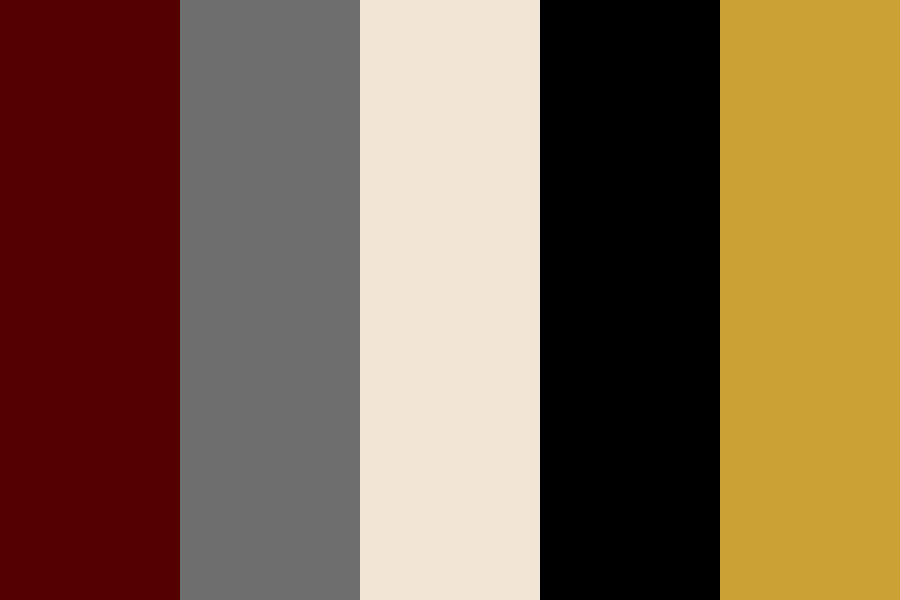The image features a minimalist design with five vertical stripes of equal width arranged horizontally across the frame. From left to right, the colors of the stripes are dark maroon, dark gray, light cream, black, and dark mustard yellow. Each stripe meets seamlessly with the next, creating a clean and uniform pattern. The overall composition resembles a flag, emphasizing the simple yet striking use of color and form.